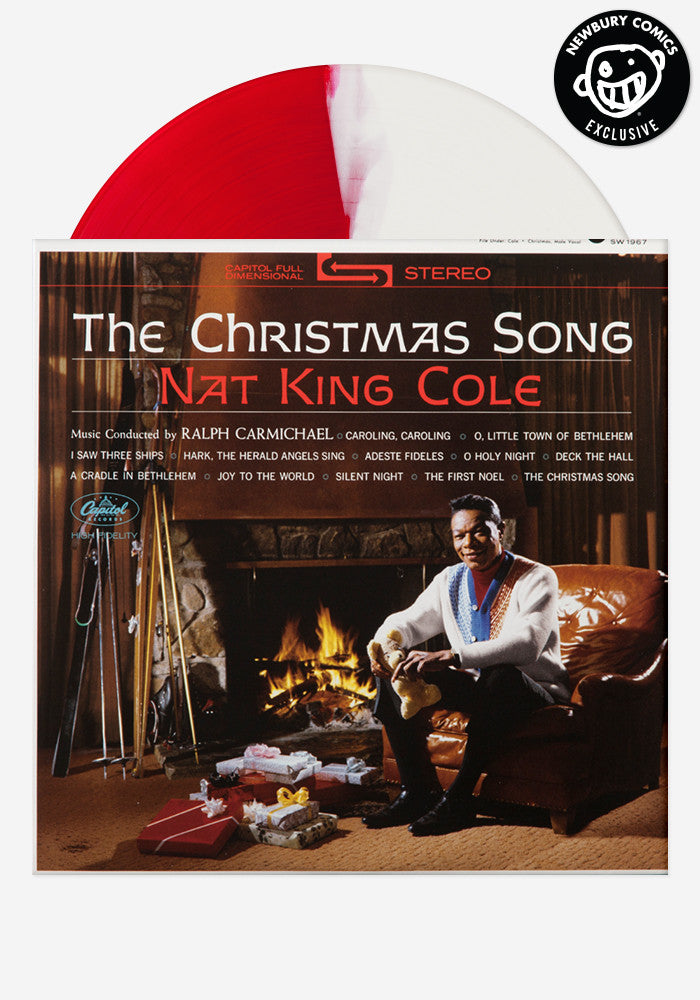This image depicts the album cover for "The Christmas Song" by Nat King Cole, released by Capitol Records. At the very top, "The Christmas Song" is written in white lettering, and just below it, notable tracks like "Caroling, Caroling," "Little Town of Bethlehem," "I Saw Three Ships," and "Holy Night" are listed. Prominently featured is Nat King Cole himself, seated comfortably on a brown leather sofa. His attire consists of a charming ensemble that includes a white knitted sweater with red accents layered over a blue shirt, and a contrasting red turtleneck underneath. The festive scene is set next to a stone fireplace with lively orange flames, adding a warm glow to the room. Surrounding him on the floor, wrapped presents add to the Christmas atmosphere. The top right of the image includes a sticker indicating it’s a Newberry Comics Exclusive. Additionally, a two-toned red and white record is part of the display, suggesting it might be part of the package or a special collector's edition.